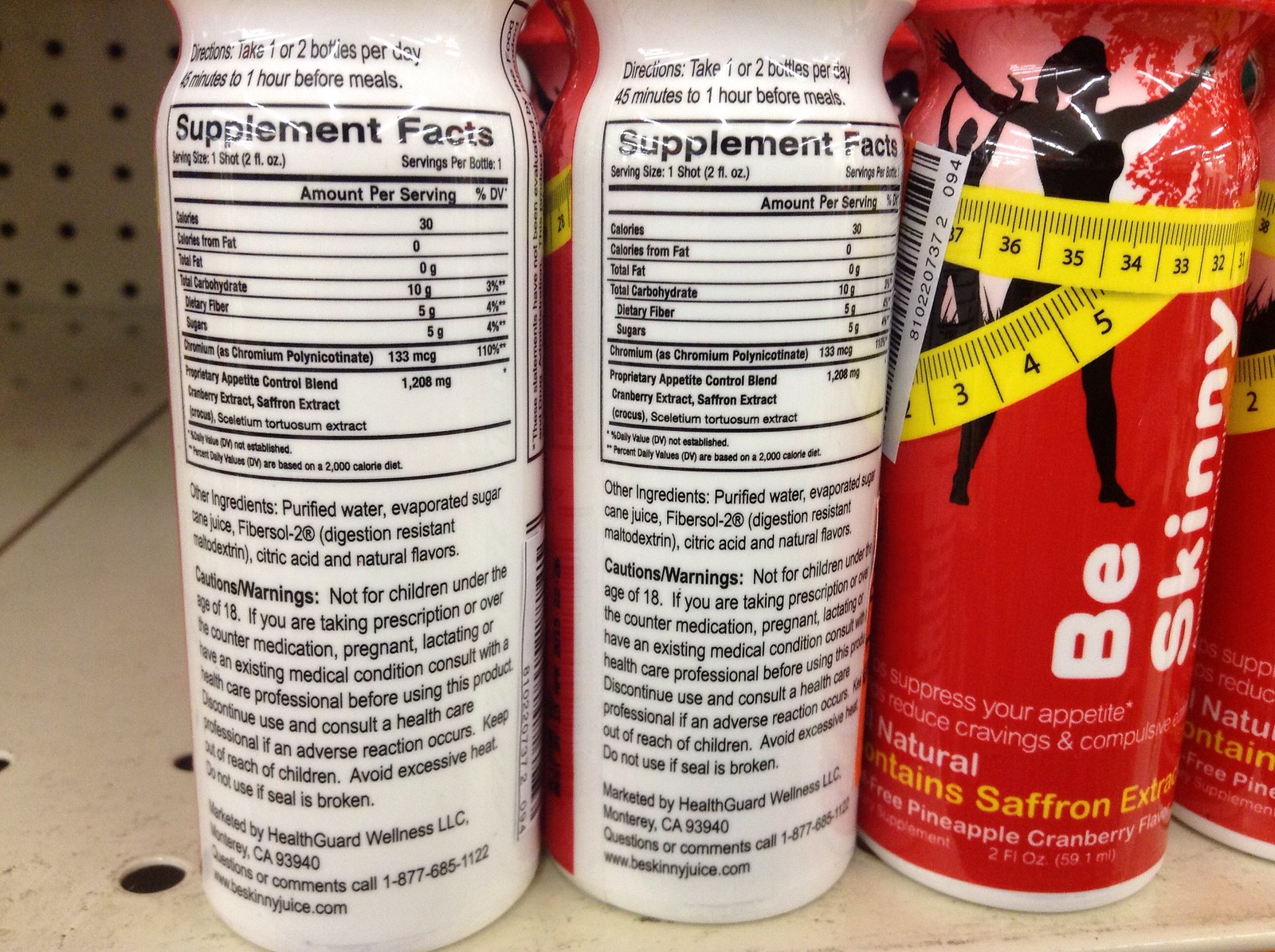This image is a detailed close-up photograph of a dietary drink product called "Be Skinny," captured on a grocery shelf. The image features two bottles of the appetite-suppressing drink: one displaying the front and the other showing the backside. The front bottle is red with white text, labeled "Be Skinny," and includes a black silhouette of a woman with her arm stretched outwards, surrounded by a measuring tape. This bottle is highlighted as being pineapple cranberry flavored and boasts natural saffron extract. The back bottle reveals the supplemental facts and nutritional information, such as calories, fiber, and carbohydrates. The label directs consumers to take one or two bottles per day, 45 minutes to an hour before meals, and includes a warning that it is not suitable for children under 18. Additionally, it advises those taking medications, pregnant, or with medical conditions to consult a healthcare professional. This product aims to suppress appetite and reduce cravings, and the photograph captures four such bottles on a store shelf.